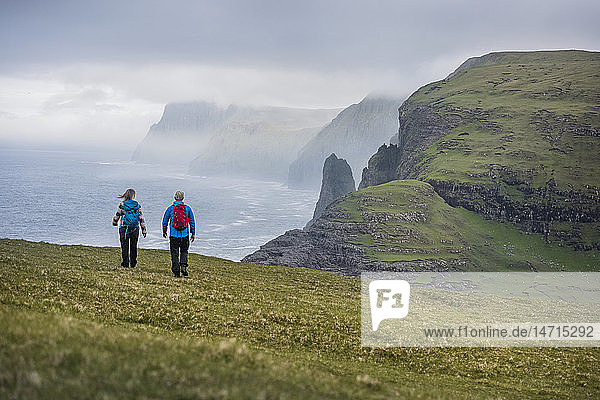This horizontal rectangular image captures a stunning landscape of a cliffside overlooking a body of water, with waves visibly approaching the land. The grassy terrain, though not wild, is covered with short green vegetation and features a sizable rock formation on the right. Two hikers, dressed in long-sleeve shirts and black pants, are seen walking away from the viewer. The man, identifiable by his long-sleeve blue shirt and red backpack, walks alongside the woman, who wears a striped shirt and carries a blue backpack. The overcast sky is filled with heavy, low-hanging clouds that obscure part of the mountainous background, contributing to the dramatic and picturesque atmosphere of the scene. In the bottom right corner, a clear gray rectangle with the letters "F" and "1" is visible.